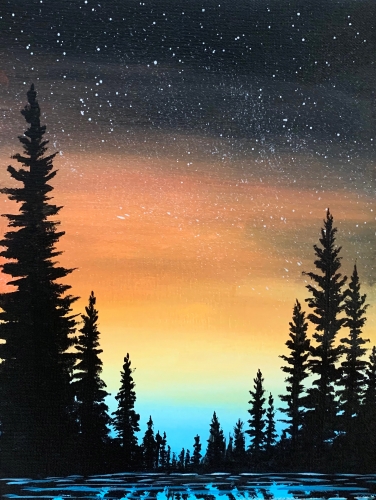"Sunset Pine Silhouette" is a captivating painting that beautifully captures the serene transition from sunset to night. Dominated by a vibrant sky that fades from amber, orange, and yellow near the horizon to deep blues and greens, and finally to the black of the night sky adorned with twinkling stars, this piece evokes tranquility. Silhouettes of tall ponderosa pine trees, reminiscent of those found in Flagstaff, Arizona, stretch across the painting, their dark forms stark against the colorful backdrop. These trees frame an opening in the center where distant blue sky is still visible. The base of the painting features what appears to be the tranquil surface of a pond or marsh, reflecting the sunset colors and the silhouettes of the pine trees, reinforcing the sense of calm and solitude. This exquisite scene artfully blends the vivid hues of a sunset with the onset of night, offering a detailed and immersive outdoor experience.